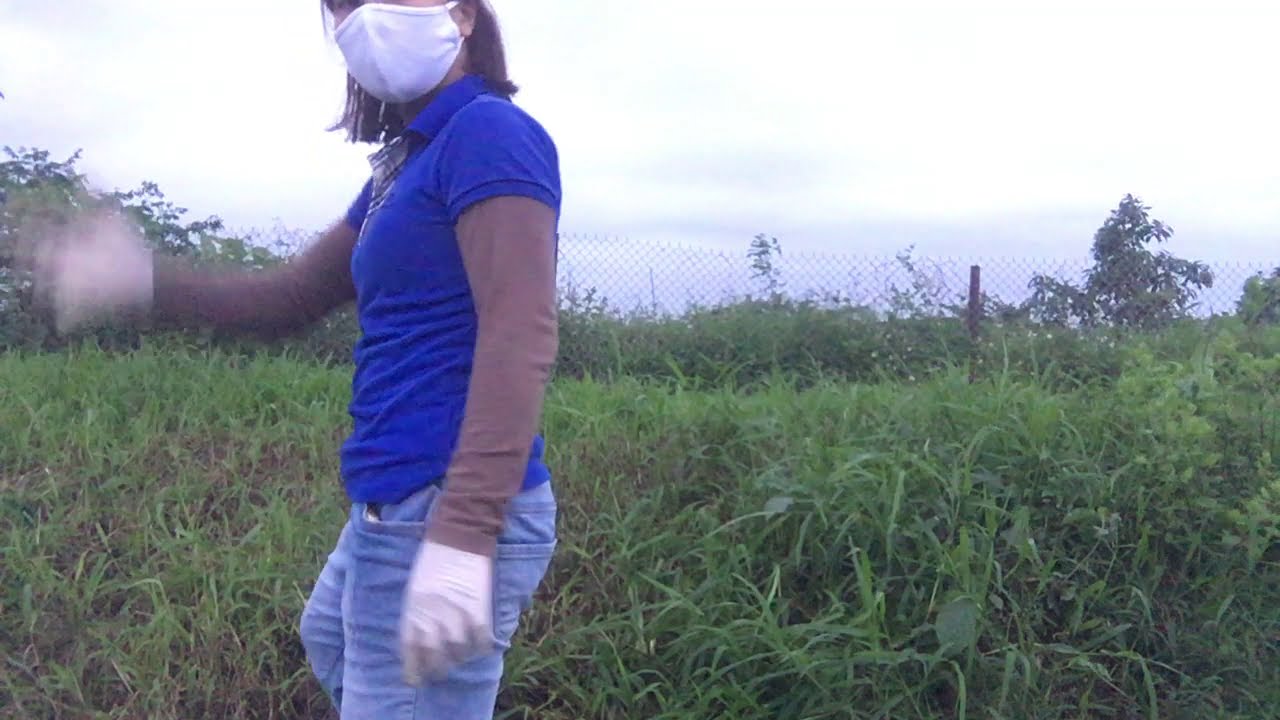In this outdoor photograph, a person with neck-length hair, wearing a blue polo shirt over a brown long-sleeve shirt, blue jeans, white gloves, and a white COVID mask, stands in a wild, grassy area. The figure, whose gender is not distinctly identifiable, is seen from the side with their left arm resting by their side and their right arm blurred in motion, possibly waving. The background features thick, natural, grass growing up to nearly two feet high, intermixed with weeds and deciduous shrubbery. The scene also includes a sagging chain-link fence, lacking its top rod, further from which a hazy, cloudy sky is visible, adding to the overall atmosphere of the wild landscape.